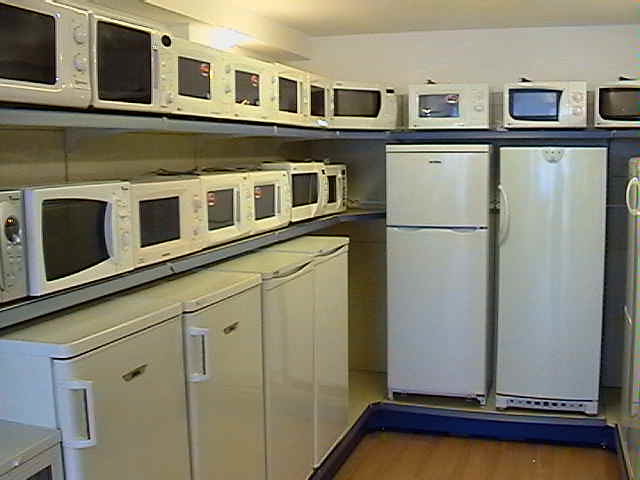The photograph captures a landscape-oriented, color image of a small kitchen appliance store's interior, albeit in low resolution. The main display forms a compact U-shaped area featuring two shelves filled with a variety of white microwaves. These microwaves, approximately a dozen in total, dominate the top shelf, displaying a variety of designs with black glass doors and a mix of control types—some featuring dials and others buttons, all located on the right side. Below, another row houses around six additional microwaves, similarly white with black fronts.

Beneath the microwaves, the bottom shelf showcases an assortment of refrigerators, seven in total, ranging in size and style. To the left, underneath the microwaves, are four dorm-sized refrigerators, characterized by either door pulls or scalloped tops to provide easy access. These compact fridges, ideal for college dormitories, align in neat, white uniformity. Directly at the end of the U-shape, there are two slightly larger, apartment-sized refrigerators raised on a small platform; one featuring a separate fridge and freezer compartment and the other a single-door unit potentially containing an internal freezer.

In addition, above these two fridges on yet another shelf, sit three more white microwaves. The store's room, painted white with brown wood flooring, includes some up lighting above the appliance displays. On the right-hand side, other appliances are partially visible, identifiable only by a handle protruding into view, hinting at a larger inventory beyond the frame.